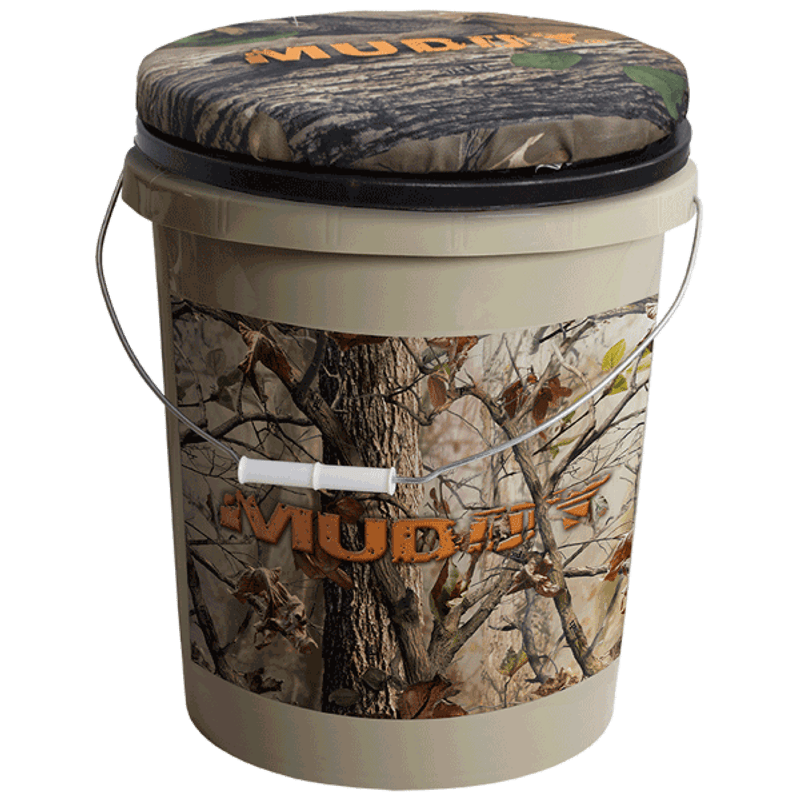The image showcases a large, camo-themed bucket, likely designed as a product for hunters or outdoor enthusiasts. The bucket itself is an off-white or grayish color and features a thin metal handle with a white plastic grip at the center for easy carrying. Prominently displayed on the side of the bucket is a rugged-looking logo in orange font that spells "MUDN" or "M.U.D.N.T," though the exact text is somewhat unclear due to a stylistic choice. Behind the logo sits an image of a tree with brown leaves, giving it an autumnal, woodsy appearance. This visual theme continues on the bucket's cushioned lid, which serves as a seat. The lid, also camouflaged, bears the same orange logo and features another nature scene, likely depicting tree bark or a woodland setting.